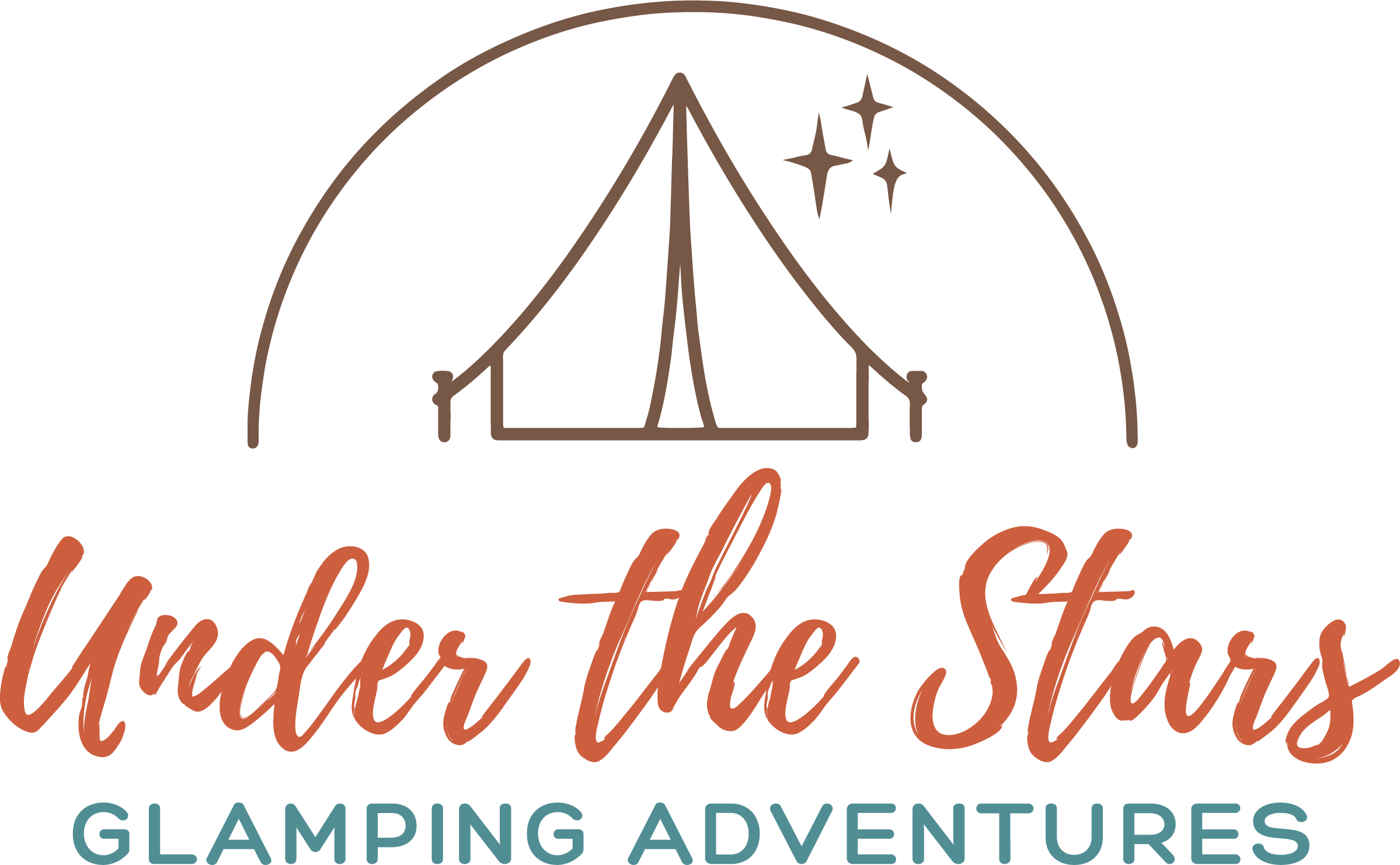The image features a logo centered on a solid white background. The logo is primarily dark brown and depicts a stylized tent. This tent features an outline with two stakes on either side at the base and an open entrance triangle extending upward. Above the tent, a brown arc forms a half-circle stretching from the left center to the right center of the image. To the upper right of the tent are three diamond-shaped stars of varying sizes. Below this illustration, the phrase "Under the Stars" is written in red cursive. Beneath this, the words "GLAMPING ADVENTURES" appear in bold, uppercase, teal sans-serif letters. The logo and text together are just over three quarters the width of the white background.